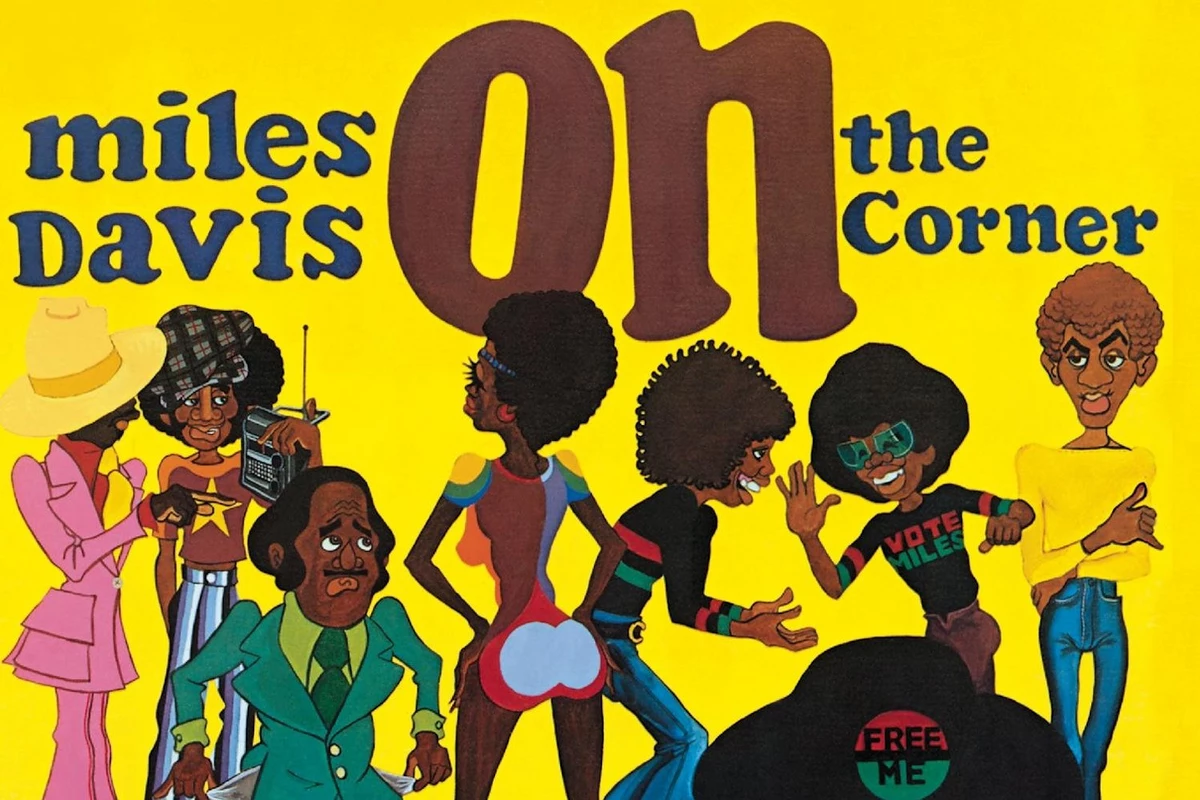This image is of a vibrant painted artwork, likely an album cover or advertisement for Miles Davis, titled "Miles Davis On the Corner" in a striking blue and brown font at the top. Set against a bright yellow background, the scene depicts seven African American caricature-style figures dressed in flamboyant 1970s disco attire, each engaged in different activities. Among them, one man stands out on the left holding a boombox, while others seem to be dancing or conversing animatedly. A prominently featured woman stands at the center, posing with an exaggeratedly curvaceous figure, and another man is seen in a green suit. One character sports a shirt that reads "Vote Miles" in a color scheme matching the pin on a wide-brimmed black hat located in the lower right corner of the image. The pin, shaded red on top and black-and-green on the bottom, carries the text "Free Me," adding a provocative touch to the dynamic and expressive tableau.